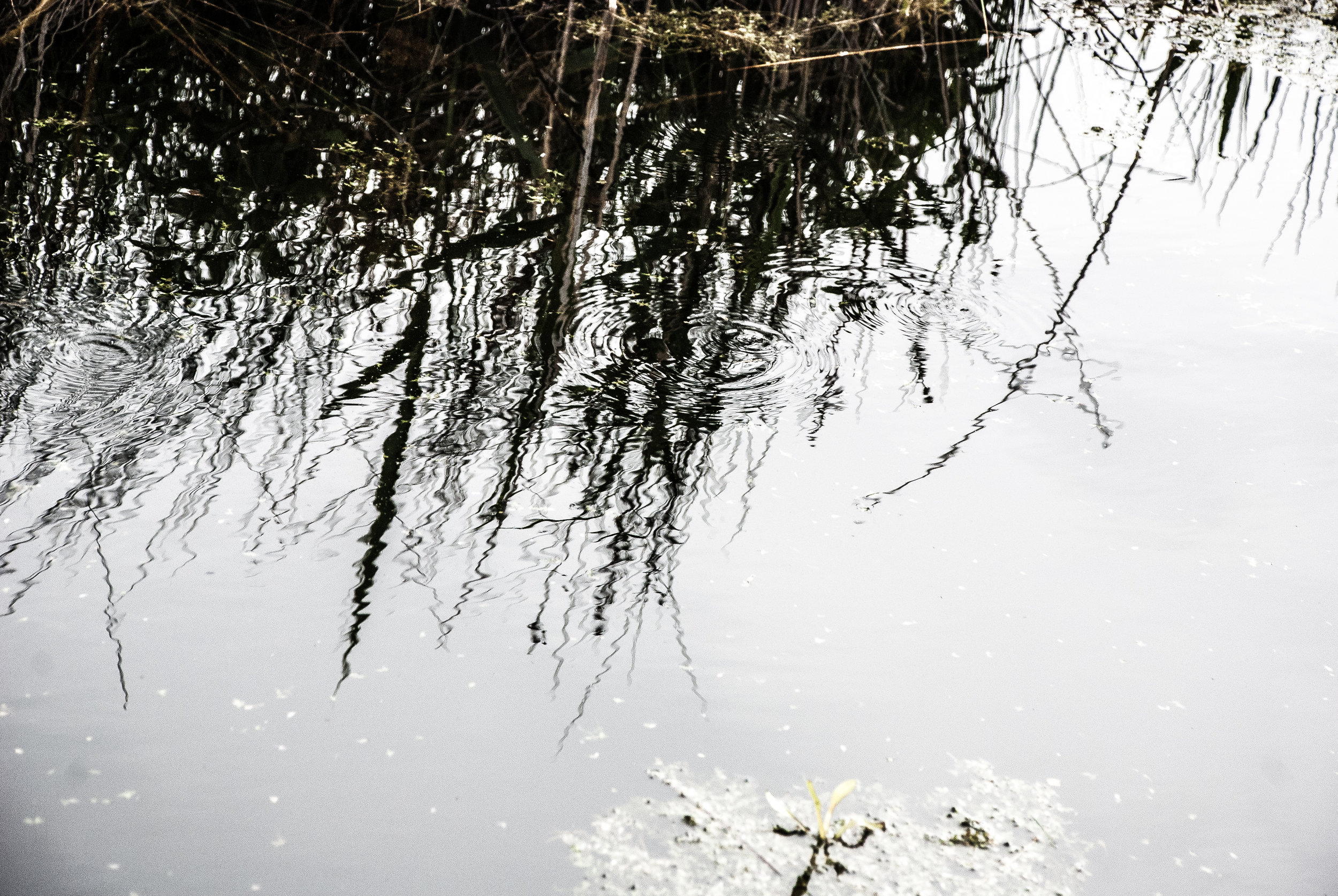This is a detailed photograph of a small pond, captured as if you're standing right at its edge and looking down. The water is somewhat murky, reflecting the overcast sky, which gives the entire scene a muted, grayish tone. The surface of the pond is adorned with gentle ripples, possibly caused by raindrops or tiny fish disturbing the water. Tall reeds and grasses, featuring fluffy, cotton-like tops, dominate the scene. Their stems and silhouettes are prominently reflected in the pond's surface along with some floating vegetation. Specifically, there's a lily floating at the bottom of the image, and spikes of reeds are visible in the top right corner. The composition and angle of the photograph emphasize the tranquil and somewhat somber beauty of this natural setting.